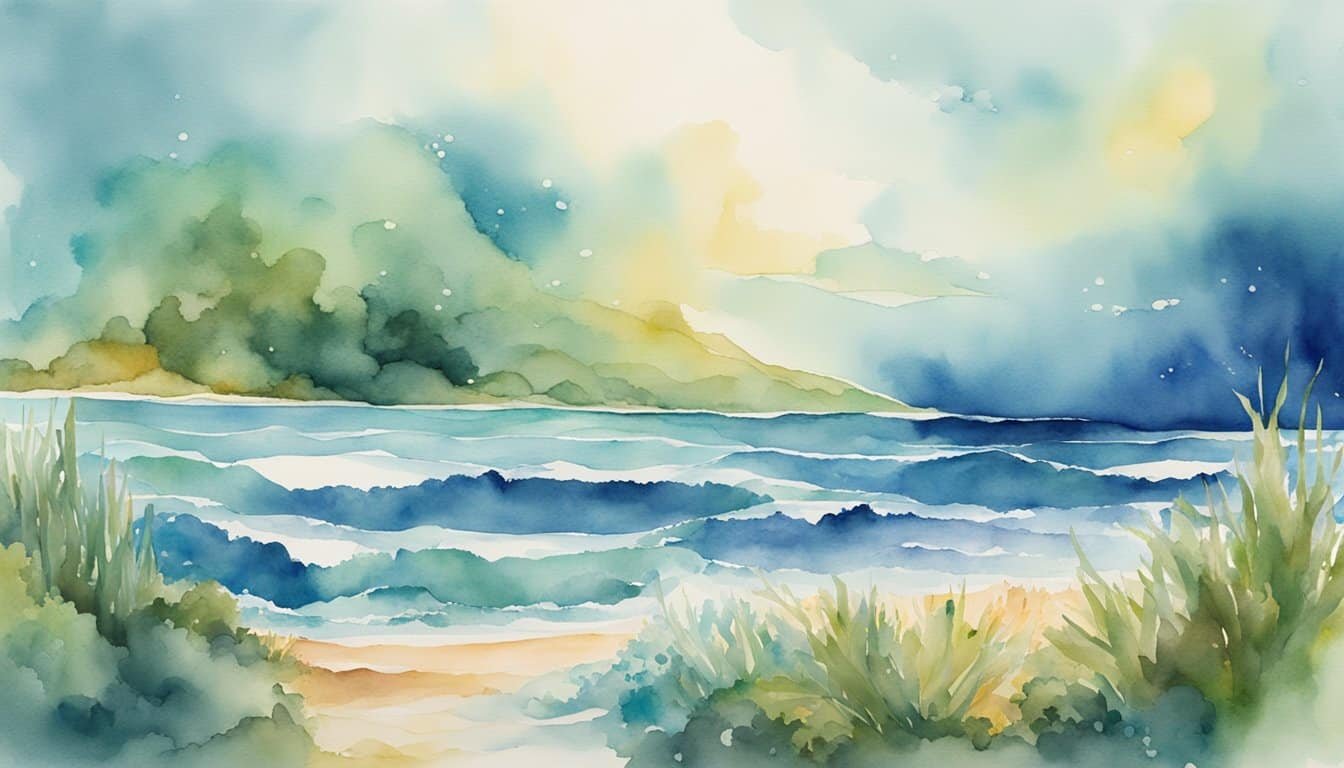This is a watercolor painting of a picturesque, deserted, small beach area. The sandy shore is light brown and dotted with small green bushes and grass, providing a quaint and serene atmosphere. Gentle waves, depicted in blue and white, lap against the shore, creating a sense of movement in the otherwise still scene. The water body, possibly a river or coastal inlet, extends across the middle of the painting, leading the viewer's eye to another island or landmass in the distance, which appears as a modest hill. The sky is a blend of cloudy whites, blues, and hints of yellow, subtly illuminated by a sun obscured by clouds. The impressionistic style of the painting causes the elements of sky and vegetation to blend softly into each other, enhancing the dreamlike quality of the landscape.